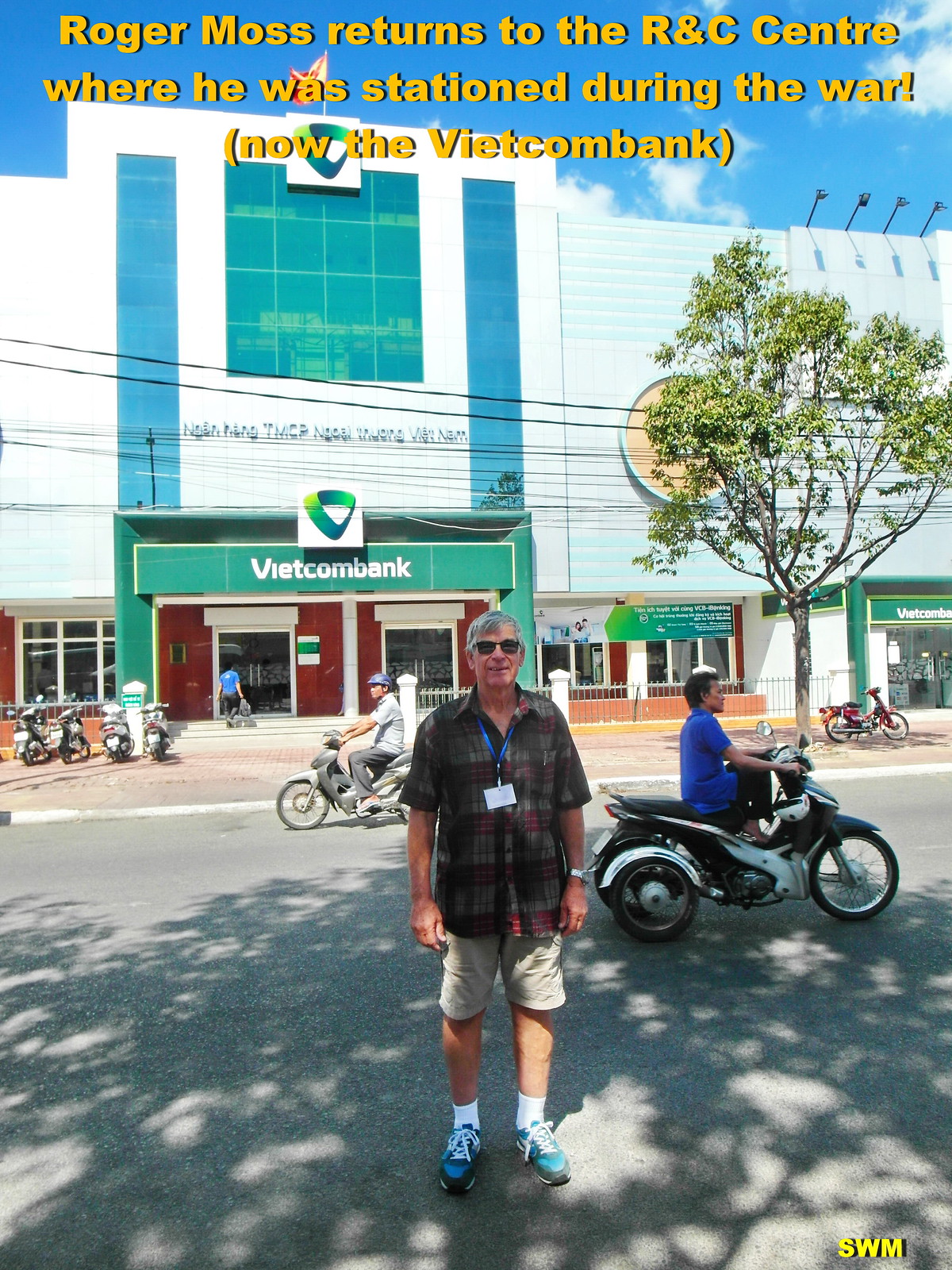In this vibrant outdoor photograph, an older Caucasian gentleman, possibly in his 60s or 70s, stands confidently in the middle of a sunny street, posing for the camera. He is dressed casually in a dark, short-sleeved flannel shirt, beige shorts, blue sneakers, and black sunglasses, with a blue lanyard around his neck. Behind him, the bustling street features a few motorcycles, some ridden and some parked, interspersed with bicycles and a trike motorcycle.

The backdrop showcases a large, imposing four-story building emblazoned with the sign "Vietcom Bank" above its multiple entrances. The building's entrance is flanked by motorcycles and a small, young tree. Adding a layer of narrative, yellow text across the top of the image reads: "Roger Moss returns to the RNC Center where he was stationed during the war. Now the Vietcom Bank." At the bottom right corner, the initials "SWM" are discreetly written. The photograph captures a mix of contemporary activity and historical reflection under a clear blue sky dotted with white clouds.